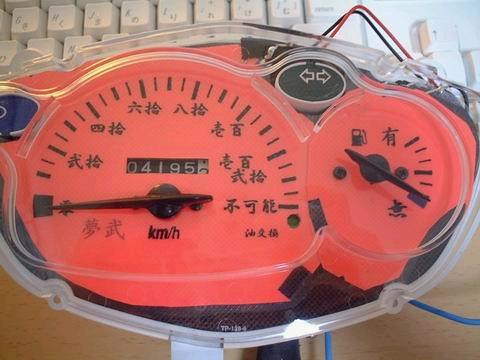The image showcases a detached speedometer held above a keyboard, with a wooden desk visible in the foreground. The speedometer is encased in clear plastic, with an orange base adding a pop of color to the design. Positioned in the top left corner is a noticeable blue button, while the primary function of the speedometer is to display speed in kilometers per hour. Surrounding the speedometer dial are markings in an Asian script, adding an exotic touch to the instrument. At the center, the odometer measures the distance traveled in standard numerical digits. Situated to the right of the speedometer is a control button marked with left and right arrows. Further right, there is a smaller gauge indicating the fuel level, complete with a gas pump icon for easy identification. The fuel gauge, like the speedometer, uses Asian characters to denote the empty ('E') and full ('F') positions.